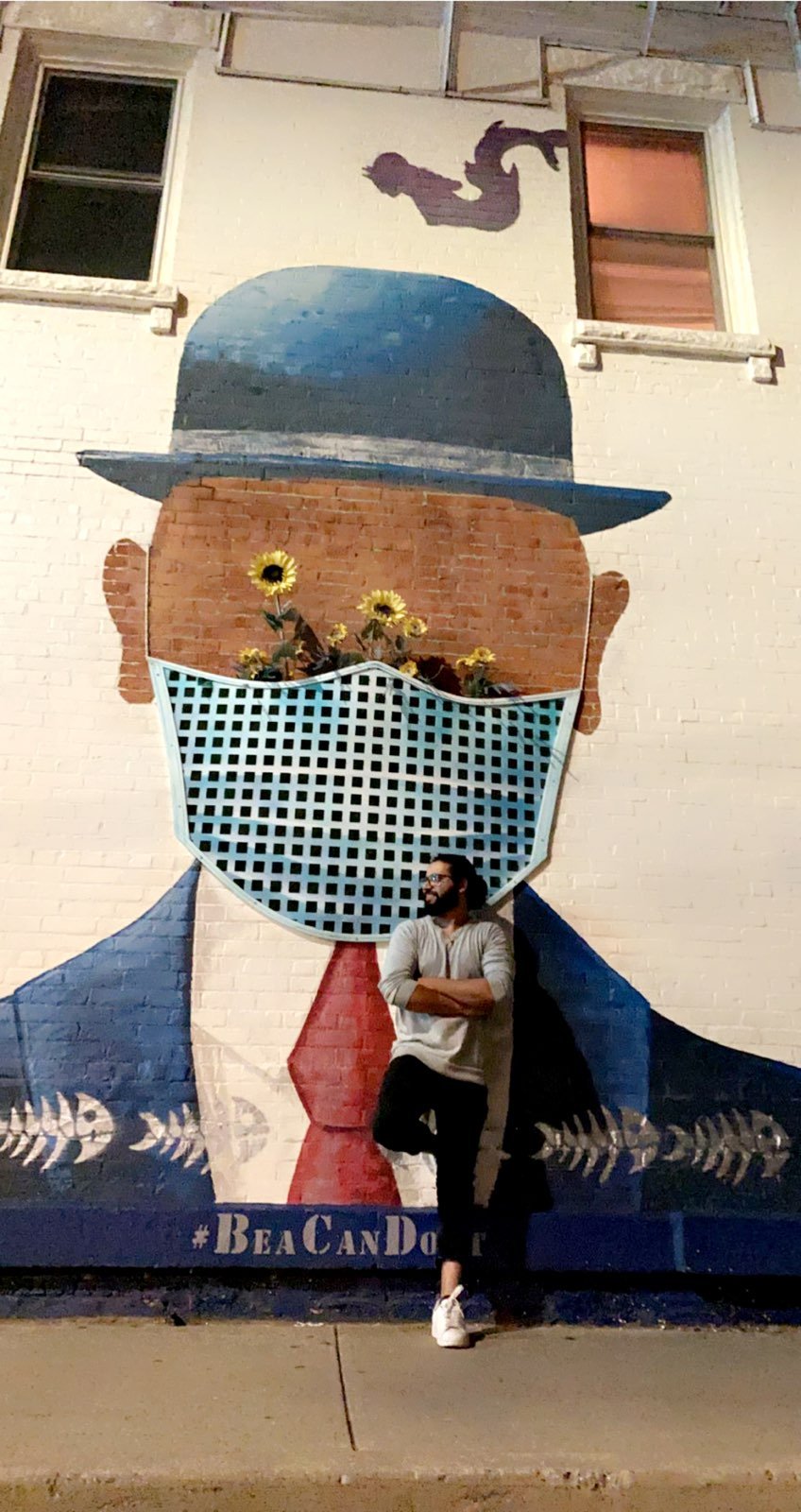The photo captures a man leaning against the outside wall of a white brick building. He is dressed in a gray long-sleeved t-shirt, black jeans or tight-fitting pants, and white tennis shoes. He has a full beard, glasses, and his hair is pulled back. Behind him is a large mural featuring a faceless man in a blue bowler hat, a blue suit, and a red tie. The mural creatively uses the underlying brown bricks from the wall to represent the face and ears of the character. The bottom half of the faceless man wears a wooden grill acting as a face mask, from which sunflowers or dandelions are growing, symbolizing a push for masks and possibly vaccinations during COVID times. Below the imagery, the text reads "#BeACanDoIt" or "#VAcanDoIt." The scene includes a sidewalk in front of the wall, and there are two windows above the mural, one illuminated and one in darkness.